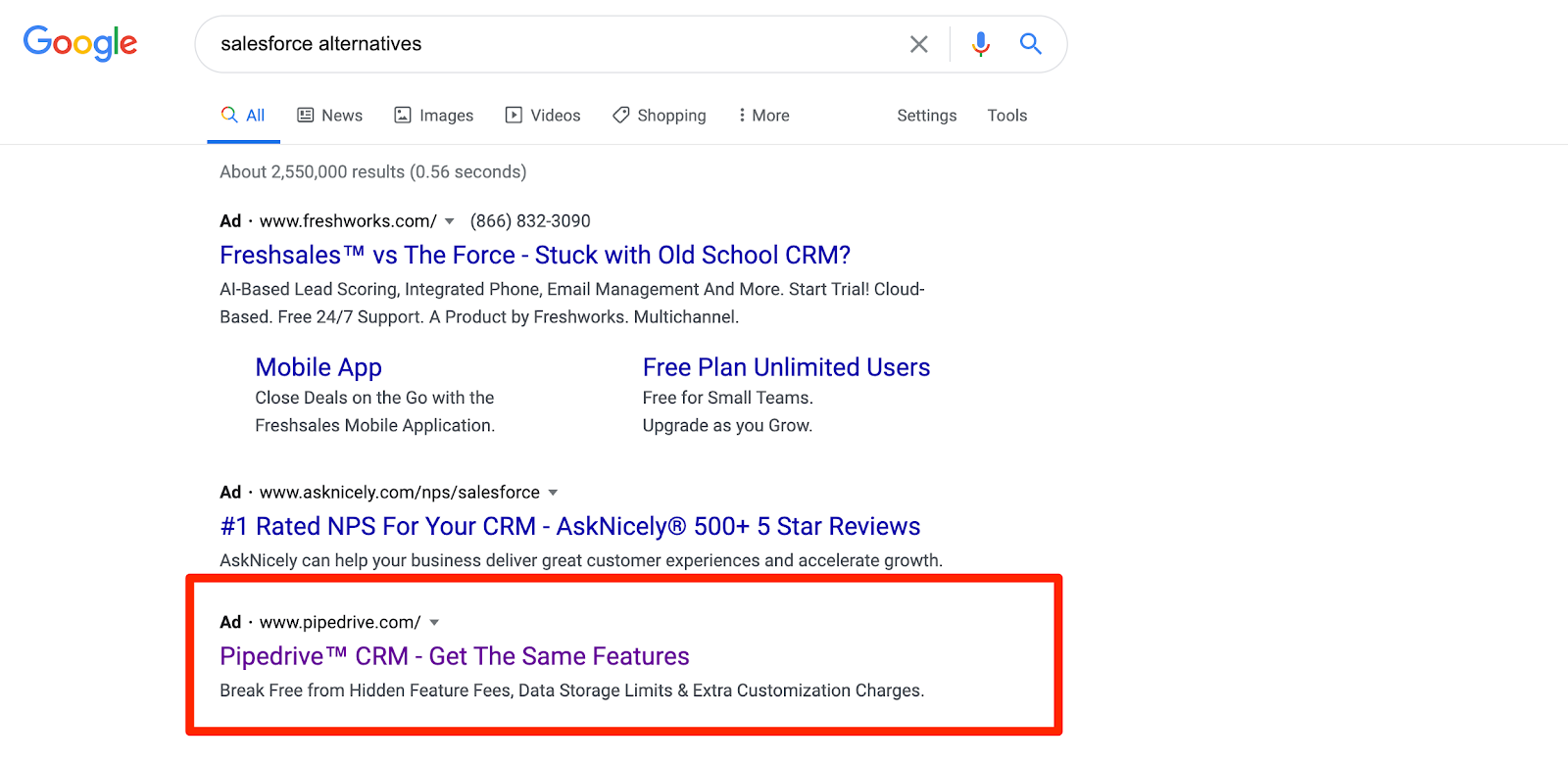The image is a rectangular screenshot from a Google search results page, set against a white background. At the top left corner, the vibrant Google logo is prominently displayed. Directly to the right of the logo is the search text box containing the query "Salesforce Alternatives."

Immediately below the search bar, navigation tabs are listed: "All," "News," "Images," "Videos," "Shopping," "More," "Settings," and "Tools." Just beneath these options, three initial results are displayed, all marked as advertisements.

The first ad titled "Fresh Sales vs. The Force," critiques traditional CRM systems, describing them as "stuffed with old school CRM." It also includes two additional links for a mobile app and a free plan, mentioning the benefit of unlimited users.

The second ad boasts being "Number one rated NPS for your CRM" and highlights "500+ five-star reviews," posing an appealing option for potential users.

The third ad stands out with a red border around it and a title in purple, indicating it has been previously clicked. The highlighted ad reads, "Pipe Drive CRM get the same features," suggesting parity in features compared to other options.

The detailed structure and visual cues in the image reflect an organized snapshot of Google search results, focusing on alternative CRMs to Salesforce.